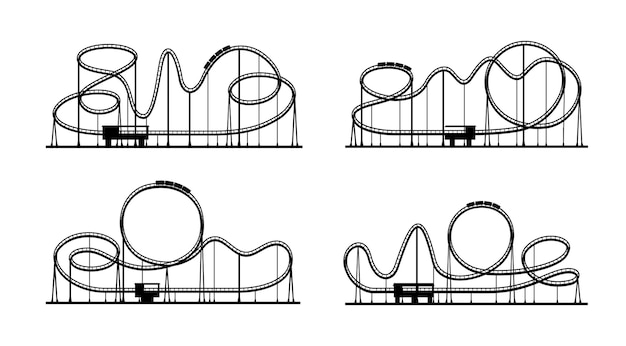The image consists of four detailed, rectangular, black and white 2D diagrams of roller coaster designs, arranged in a grid with one in each corner: top left, top right, bottom left, and bottom right. All four layouts exhibit unique structures but share significant features, such as loop-the-loops and corkscrews, depicted with intricate trajectories.

The first roller coaster features figure-eight patterns, several steep drops, and a loop. The second design showcases a prominent central loop, accompanied by smaller drops and a corkscrew element. In the third roller coaster diagram, a massive loop is positioned in the middle, preceded by small hills, followed by a corkscrew. The fourth illustration starts with a corkscrew, leading into a substantial loop, a steep descent, and a hill that curves to the left.

Each roller coaster shows four small cars on the tracks, although no passengers are depicted. Below each ride, a station of varying sizes, ranging from very small to considerably larger, is illustrated for loading and unloading passengers. The designs are either digitally rendered or hand-sketched, highlighting the versatility and creativity in roller coaster engineering.